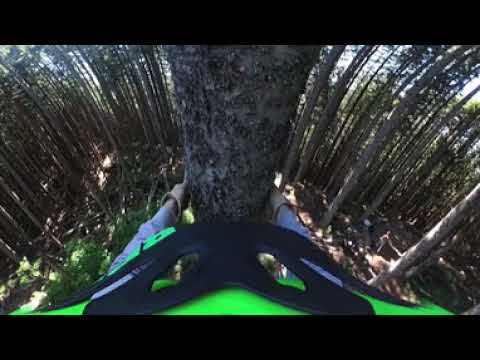This photograph captures a surreal forest scene dominated by tall, slender tree trunks that are mostly bare of branches and leaves. Central to the image is a tree of medium diameter, about 12 inches, being embraced by a person who appears to be climbing it. The climber is adorned in a light blue long-sleeved shirt and brown gloves, their arms wrapped securely around the tree. The individual also wears a black harness, partly visible along with a bright green shirt or equipment piece. The lower part of the image is marked by the thick black borders at the top and bottom, adding a dreamy, distorted ambiance to the overall scene. The surrounding forest is filled with similarly narrow trees, which curve slightly and let in patches of sky and sunlight, casting intricate shadows across the forest floor where sparse greenery and weeds grow.